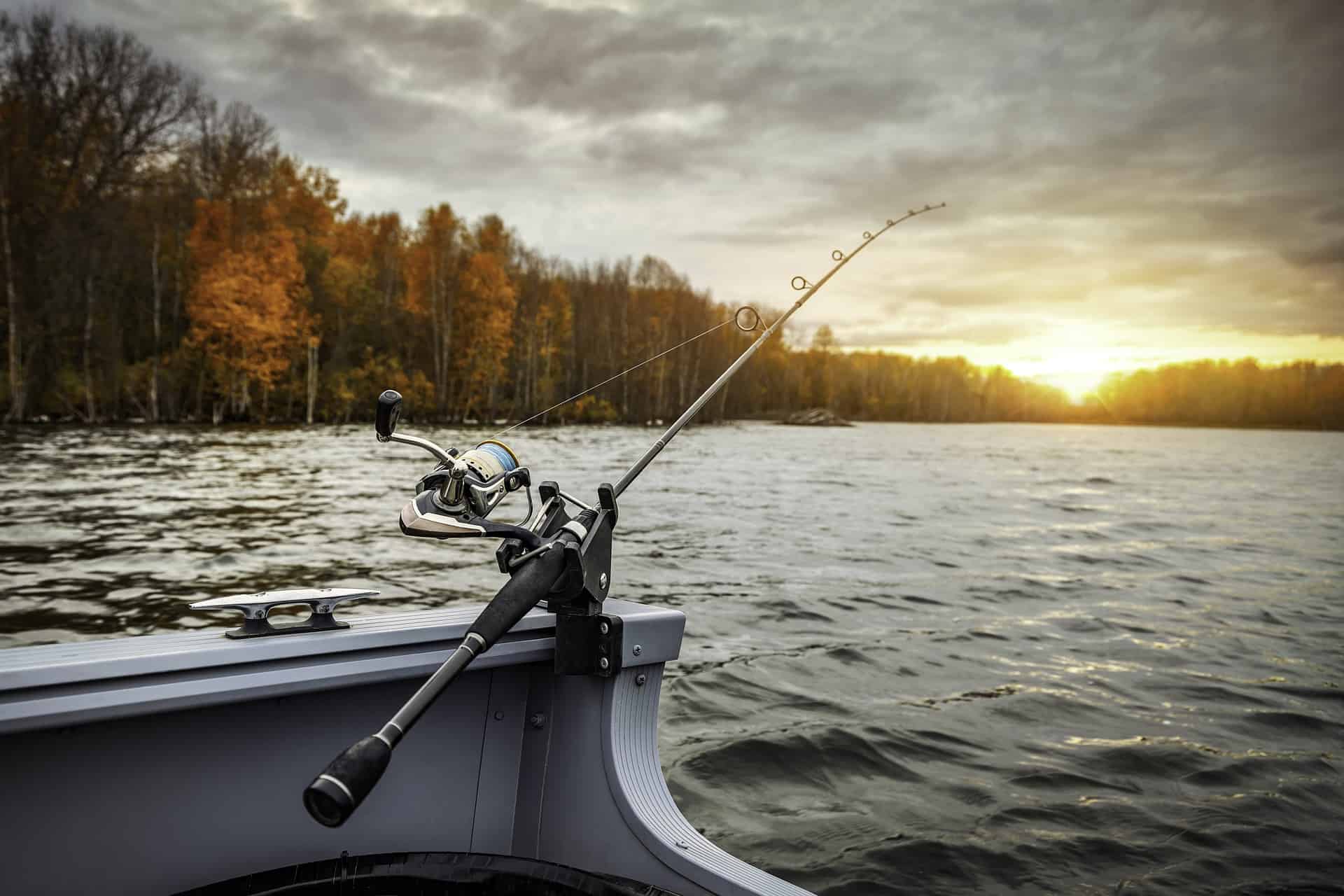The image depicts a grey, metal fishing boat, specialized for fishing activities. Mounted on the corner of the boat is a robust black fishing rod, securely screwed into the structure. The fishing reel attached to the rod is a metallic silver with a black knob on the handle, suggesting durability and readiness for use, as the line appears to be cast already. Adjacent to the fishing rod, on the left side, there's a chrome tie-down. The backdrop showcases a serene lake with slightly rippled water, flanked by trees lining the horizon on the left. On the right side of the image, the sun is either rising or setting, casting a glow over the scene. Above, dark rain clouds loom ominously, hinting at impending rainfall. No people are visible in the frame, focusing the viewer's attention on the solitary fishing rod and the tranquil, yet slightly foreboding, natural setting.